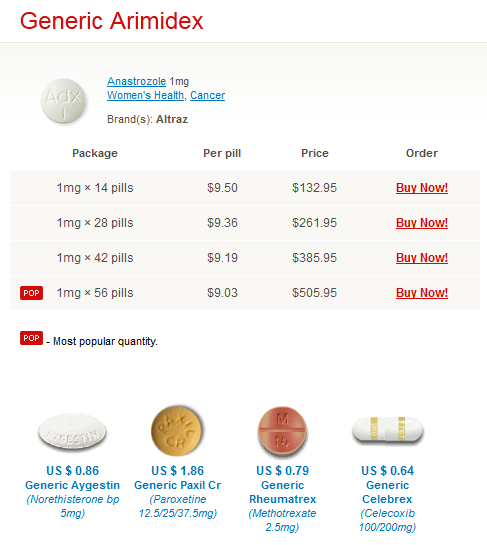Screenshot Description of a Drug Information Website:

The screenshot captures details from a website featuring information about a generic medication called Arimidex. At the top of the page, the title is prominently shown as "Generic Arimidex," with the word "ARIMIDEX" spelled out in capital letters.

Beneath the title, there is a small box displaying an image of the pill. The pill is round, white, and embossed with the characters "ADX" followed by a horizontal line. Adjacent to the image, in blue clickable text, it reads "anastrozole, 1mg." Further clickable links in blue text include "Women's Health" and "Cancer."

Listed under "Brands", the name "Altraz" is mentioned.

The bulk of the page consists of a detailed table with four columns: Package, Per Pill, Price, and Order. The table lists four different purchasing options for the 1mg dosage of the pills:
1. **1mg x 14 pills:** $9.50 per pill, total price $132.95 - Order option: "Buy Now"
2. **1mg x 28 pills:** $9.36 per pill, total price $261.95 - Order option: "Buy Now"
3. **1mg x 42 pills:** $9.19 per pill, total price $385.95 - Order option: "Buy Now"
4. **1mg x 56 pills:** $9.03 per pill, total price $505.95 - Order option: "Buy Now" (Highlighted with a red box reading "POP", indicating this is the most popular quantity)

At the bottom of the page, there are images and prices of four additional pills shown as potential alternatives or related medications:
- **White oval pill:** US $0.86, generic Agiston
- **Yellow pill:** US $1.86, generic Paxil
- **Reddish pill:** US $0.79, generic Rheumatrex
- **White capsule with gold bands:** US $0.64, generic Celebrex

Each alternative medication is listed with its medical name and dosage information.